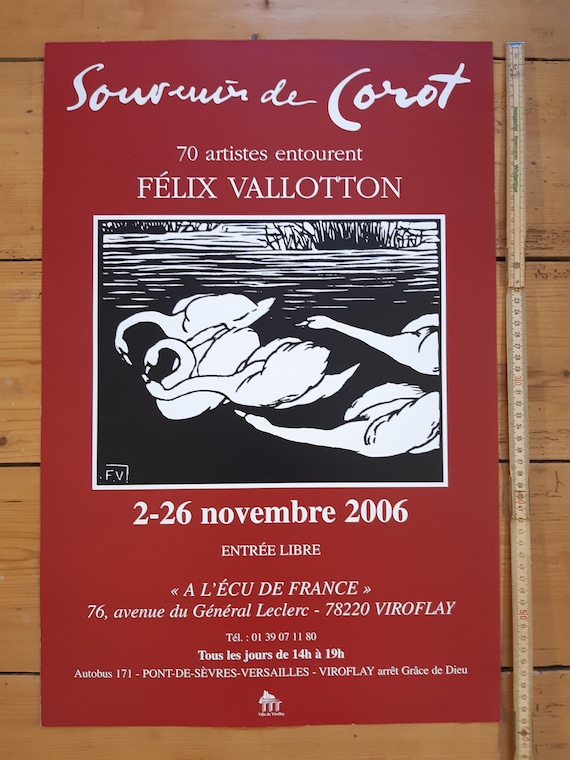The image is a photograph of a dark red, burgundy-tone poster or pamphlet, resting on a wood-planked table. To the right of the pamphlet is a measuring stick, although the details on it are not clear enough to discern the measurements. The cover of the pamphlet features a centrally located black and white lino-cut print depicting five swans on a black ocean pond. Two of the swans have their necks entangled, while the other three stretch towards the entwined pair. The text on the pamphlet is written in white and is entirely in French, detailing event information, titles, a date (2-26 November 2006, likely referencing an event timeframe), and phrases such as "Entree libre," indicating free entry. The text includes an address, possibly in Versailles, France, and a telephone number.